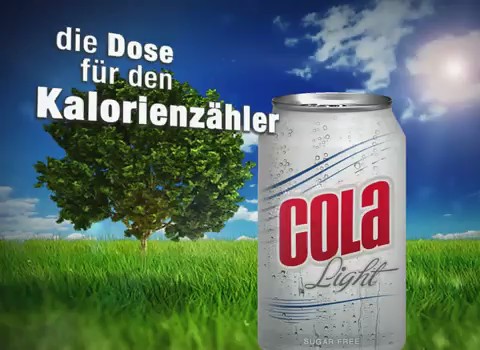This image features a meticulously Photoshopped scene that showcases a bottle of German Cola Light. The focal point is the bottle itself, prominently displayed at the center of the composition. The bottle’s label is clearly visible, with the text "sugar-free" inscribed at the bottom. It retains the iconic red color in its header, with "Light" written underneath.

The background is a surreal blend of nature, featuring a tree and a field of long grass, all set under a sunny sky. The sun is partially obscured by clouds, casting a softly diffused light across the scene. Suspended above the tree is a German inscription or possibly a slogan, adding a local touch to the image.

The edges of the image are intentionally shaded darker, creating a vignette effect that draws the viewer’s attention more towards the vibrant and highlighted center, where the Cola Light bottle stands out against its whimsical backdrop. This well-crafted digital composition not only emphasizes the product but also adds an artistic touch that makes the scene visually engaging.